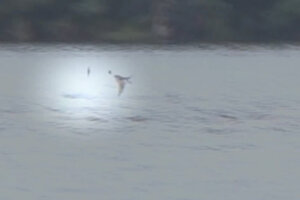The image is an extremely small, blurry, and grainy photograph, making it difficult to discern precise details. Predominantly, it features a body of water that occupies most of the frame, characterized by a light gray-blue color with some ripples, suggesting calmness. In the foreground, there is a noticeable, bright circular reflection on the water, likely indicating moonlight given the overall darkness of the scene.

Above this reflection, a bird, possibly a duck, is faintly visible in flight. In front of the bird, there might be another bird or potentially a fish leaping from the water, although these details are very indistinct and appear as dark smudges. The background of the image is notably dark and blurry, with hints of what could be a forest or shoreline, featuring vague green, black, and brown shapes that suggest trees or possibly buildings. Overall, the photograph is hazy, making the separation between the water and the background barely perceptible and leaving the intricate details largely open to interpretation.